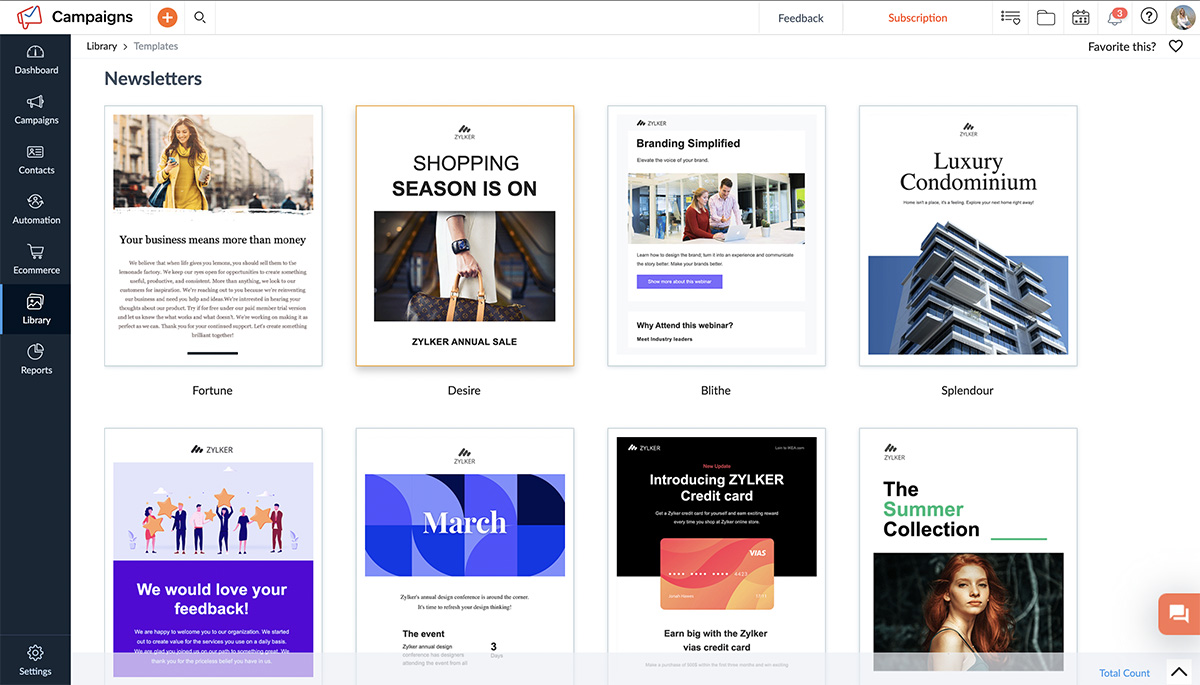In this image, the user interface is depicted in a structured manner with multiple elements neatly organized. 

In the top left corner, there is a section labeled "Campaigns" accompanied by an orange button. Directly opposite, in the top right corner, there are several icons and options including "Feedback," "Subscription," a profile icon, a notification icon, a help icon, a calendar, a folder, and a list view.

On the left side of the interface, a dark blue sidebar labeled "Sitemain" contains a menu in list format. From top to bottom, the menu items are: Dashboard, Campaigns, Contacts, Automation, E-commerce, Library, Report, with "Library" being the currently selected section.

In the main content area, eight templates are displayed under the heading "Newsletters." 

1. The first template, located in the top left corner, features an image of a woman wearing all yellow, carrying a coffee cup and a black bag, with the text "Your business need more than anything" and a blurry description beneath it.
    
2. To the right of the first template, the second template, which is currently selected, states "Shopping is on" and "Zylka annual sale." It includes an image of a man holding a Louis Vuitton bag and is outlined in orange.

3. The third template, "Branding Simplified," encourages the viewer to attend a webinar by Blit.

4. The fourth template, "Splendor," promotes a luxury condominium with an image of buildings.

5. In the bottom left, the fifth template solicits feedback with the text "We would love your feedback" against a purple background, black text, and animations of people holding yellow stars.

6. The sixth template, "Match the Event," has a blue and dark blue background with white and black text.

7. The seventh template, "Introducing Zylka Credit Card," promotes earning with the Zylka credit card. The card is depicted in yellow and orange, set against a black background.

8. The eighth and final template, "The Summer Collection," features a woman with brown hair in a forest setting. "Summer" is written in green, "Collection" in black, and the background is white.

Each template is visually distinct, with varying colors and themes catering to different campaigns and purposes.